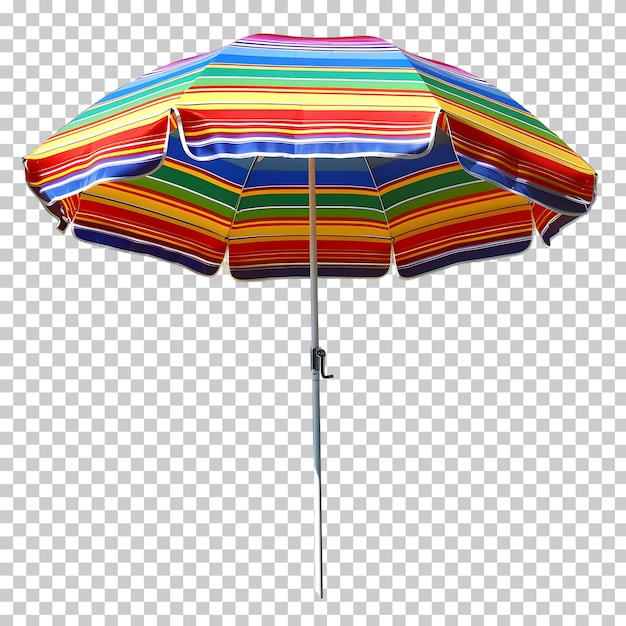This image showcases a vividly detailed, rainbow-colored beach umbrella, fully opened and standing tall at the center. The umbrella is propped up by a silver metal stem featuring a crank mechanism for adjusting the canopy. The canopy displays an array of bright colors arranged in stripes—red, yellow, orange, green, blue, and purple, with occasional white stripes accentuating the other hues. Each segment of the umbrella is supported by the central post, which extends all the way up to maintain the structure and offer protection against the wind. A subtle ruffle decorates the lower edge of the canopy. The background consists of a white and gray checkerboard pattern, reminiscent of a PNG transparency grid, which serves to highlight the umbrella's vibrant colors. The intricate illustration is so meticulously rendered that at a glance, it could be mistaken for a photograph.